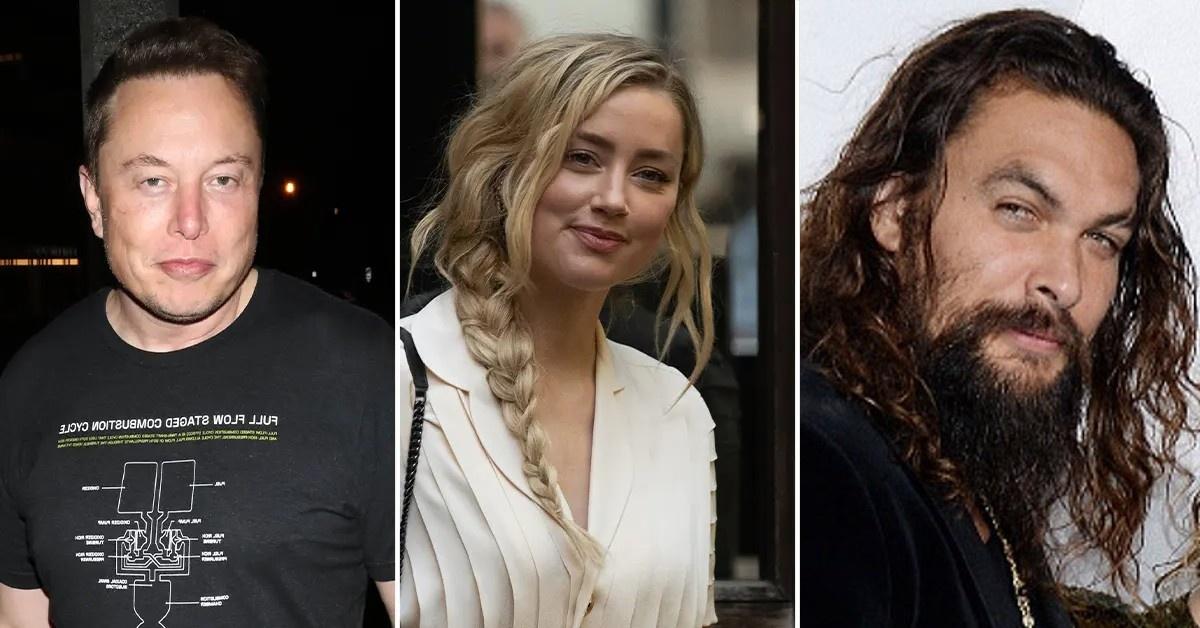The image is a horizontal collage comprising three close-up, color photographs of celebrities, each in a vertically long rectangle and separated by thin vertical white strips. From left to right, the first photograph features Elon Musk, the CEO of Tesla, who is captured wearing a black shirt with a white circuit board pattern and text, though it is unreadable. He has short dark brown hair and is set against a black background illuminated by lights. He sports a subtle smirk.

The center photograph showcases Amber Heard, the actress, dressed in a light, ruffled, beige V-neck dress coat. Her dark blonde hair is partly braided, and she's wearing red lip gloss, also flashing a slight smirk. The background behind her is blurred, suggesting depth.

The last photograph features Jason Momoa, an actor, with long, wavy hair cascading to his chest, a mix of dark brown and lighter tips. He has a beard, goatee, and mustache, all dark black, paired with a black jacket and a gold chain. His complexion is darker, likely reflecting his partial Samoan heritage. His expression is also a mild smirk, and the side view of his head is captured, adding a distinct angle to his appearance in the collage.